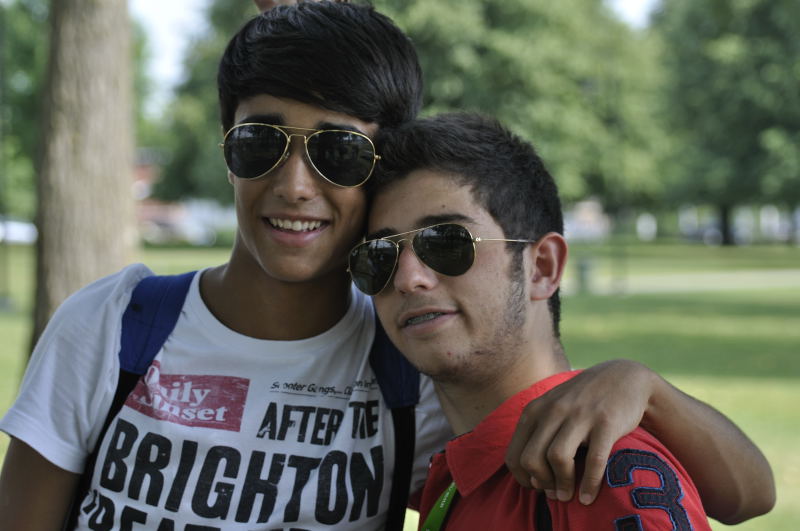In this image, two young men, likely in their late teens or early twenties, stand closely together outside, set against a blurred background that suggests a city park with a grassy field, various trees, and a walking path. The young man on the left, who has his arm affectionately around the other, sports a combed-over hairstyle reminiscent of an old Justin Bieber look. He has dark aviator sunglasses with gold frames and is wearing a white t-shirt with a design resembling a newspaper article, featuring the words "The Daily Sunset" and a headline with the word "Bright" visible. He carries a blue backpack, identifiable by the shoulder straps. His friend on the right also has dark aviator sunglasses and wears a red, rugby-style polo shirt with the embroidered number 3, outlined in blue and black, on the shoulder. This friend, who has short black hair and a bit of stubble around his chin, is wearing a green lanyard and has braces. Both are smiling, though the young man on the left has a broader smile. They appear to be enjoying a sunny day together in a park setting.